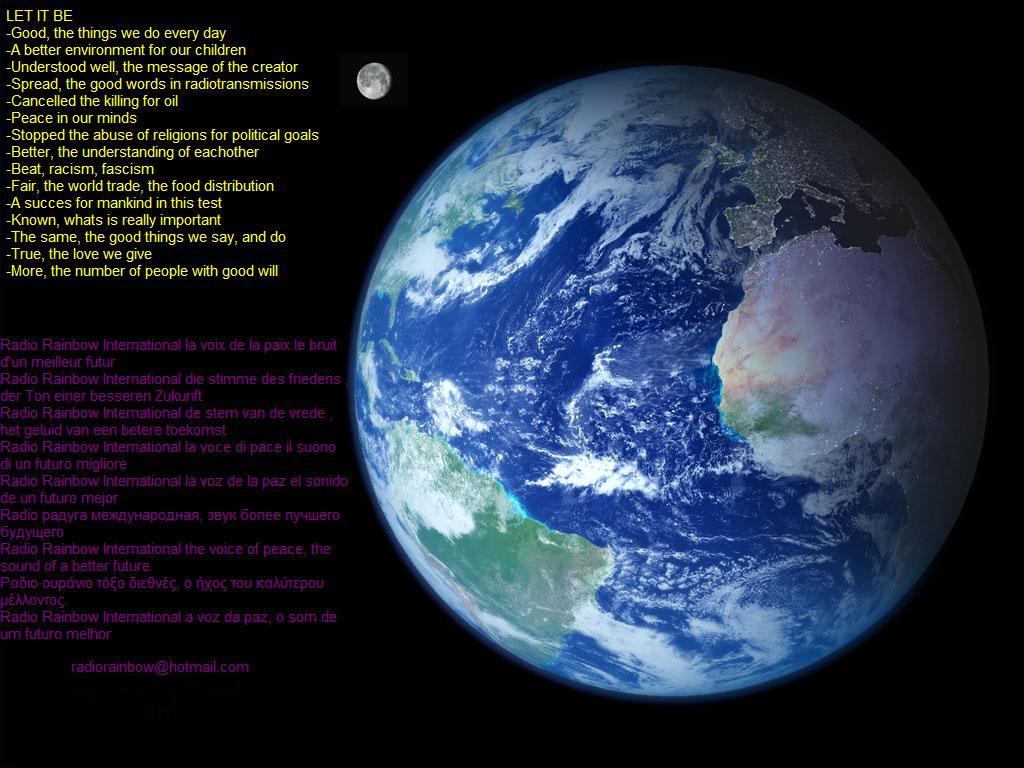The image showcases a photograph of Earth, prominently positioned on the right side with the upper left featuring the moon. The Earth appears vibrant, displaying distinct blue oceans and varied landmasses in green, brown, and some orange, resembling a detailed marble. The planet's right side is cloaked in shadow, suggesting a light source from the left.

On the left side of the image, two sections of text are present: an upper section in yellow font and a lower section in purple font, which repeats the yellow text content in French. The yellow text begins at the top with the phrase "LET IT BE" in all capitals, followed by several dash-pointed statements that outline an inspiring message:

- Let it be good the things we do every day
- A better environment for our children
- Understood well the message of the Creator
- Spread the good words in radio transmissions
- Cancel the killing for oil
- Peace in our minds
- Stop the abuse of religions for political goals
- Better the understanding of each other
- Beat racism, fascism
- Fair the world trade, the food distribution
- A success for mankind in this test
- Known what is really important
- The same, the good things we say and do
- True love we give
- The more number of people with goodwill

This comprehensive and visually rich image conveys a profound message of peace, understanding, and collective betterment, skillfully blending a stunning depiction of Earth from space with an evocative textual exhortation.